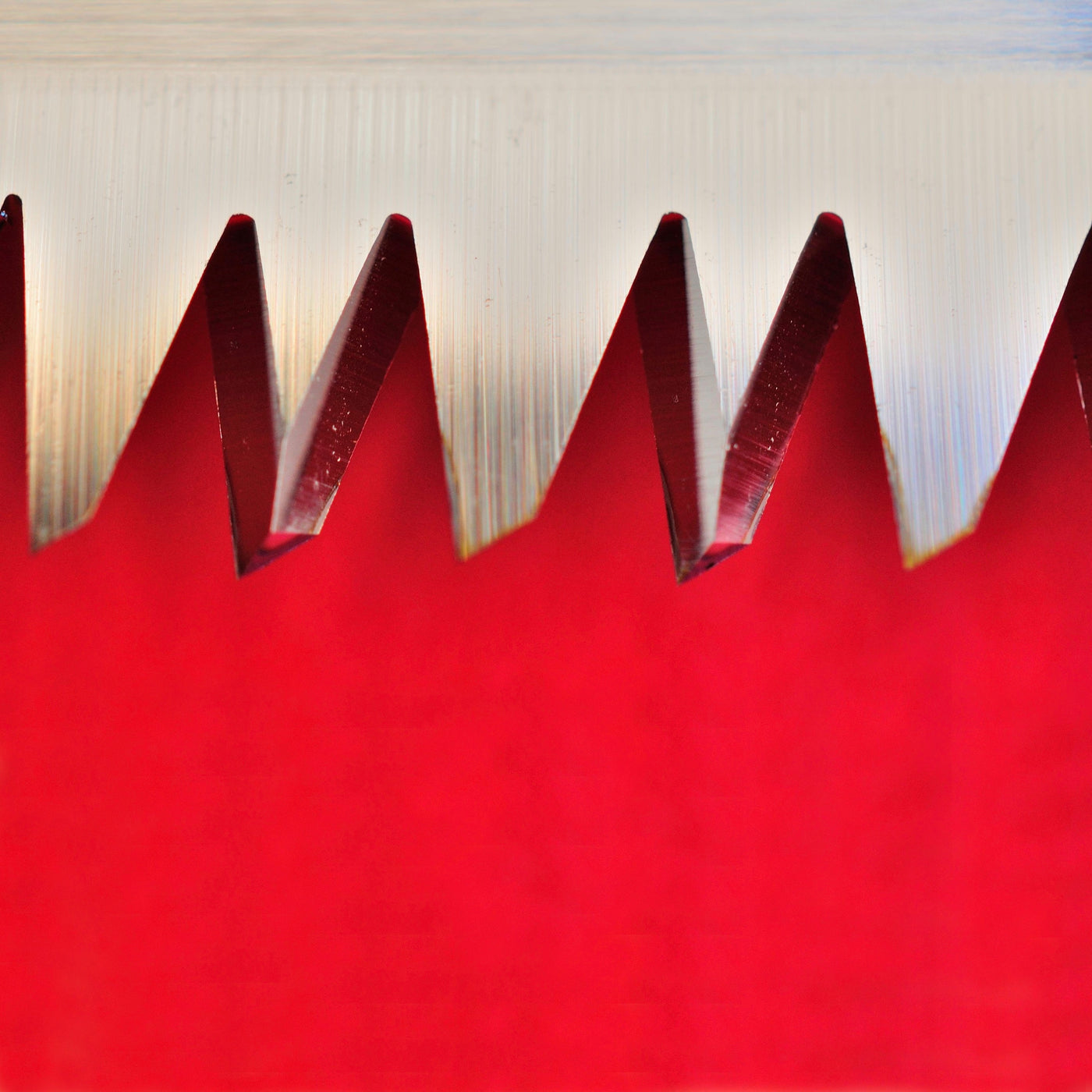This image features a close-up view of a striking, serrated red object occupying the bottom two-thirds of the frame. The object showcases four complete triangular teeth, with half of an additional tooth visible on each of the frame's edges, creating a jagged, comb-like appearance. The teeth are not symmetrical, and some spacing variations add to the irregularity of the pattern. The teeth have sharpened sides and exhibit a gradation of shades, with the tops appearing lighter and darkening towards the base. Above the red object is a striated, off-white or grayish-white surface with vertical lines, partially visible against a slightly darker solid light gray backdrop. The overall background includes a gradient from lighter at the top to darker shades moving downward, contributing to the image's intricate texture and color contrasts.